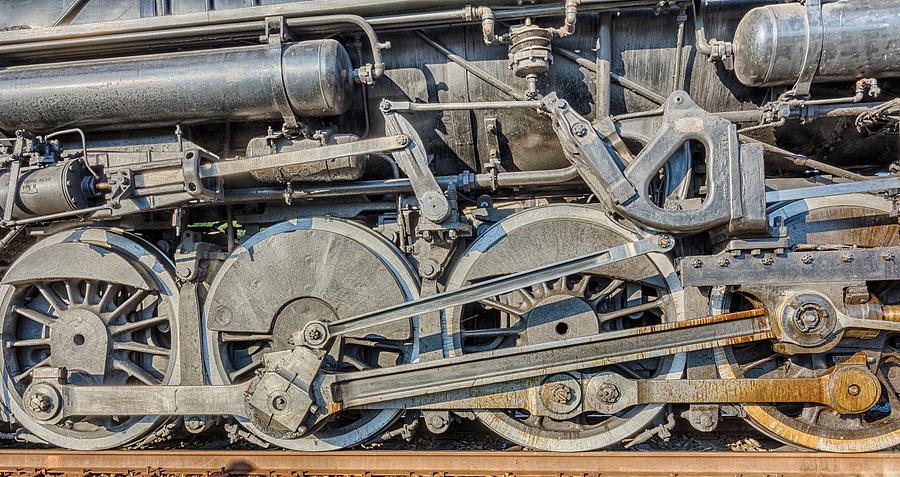This detailed, close-up photograph captures the side of a steam train engine, emphasizing four prominently displayed wheels connected by a large mechanism resembling wrenches. Approximately two feet above the wheels, several short levers, bars, and varying cylinders can be seen, some of which have hoses attached that run along a horizontal strip. The cylinders above the wheels are about five feet long and as thick as a watermelon. The engine appears old and neglected, with rust originating from multiple spots, particularly accentuated on the right-hand side. The train, which likely once had a black exterior but now hosts a predominantly gray hue, looks dusty and stained, suggesting it has either been on a long journey without cleaning or is currently inactive on the track. Visible traces of liquid stains and grime add to the weathered appearance. Despite the image showing the train during daylight, the top and ends of the train remain out of view, keeping the focus tightly on the intricate, grimy details of the wheels and mechanical structures just above them.